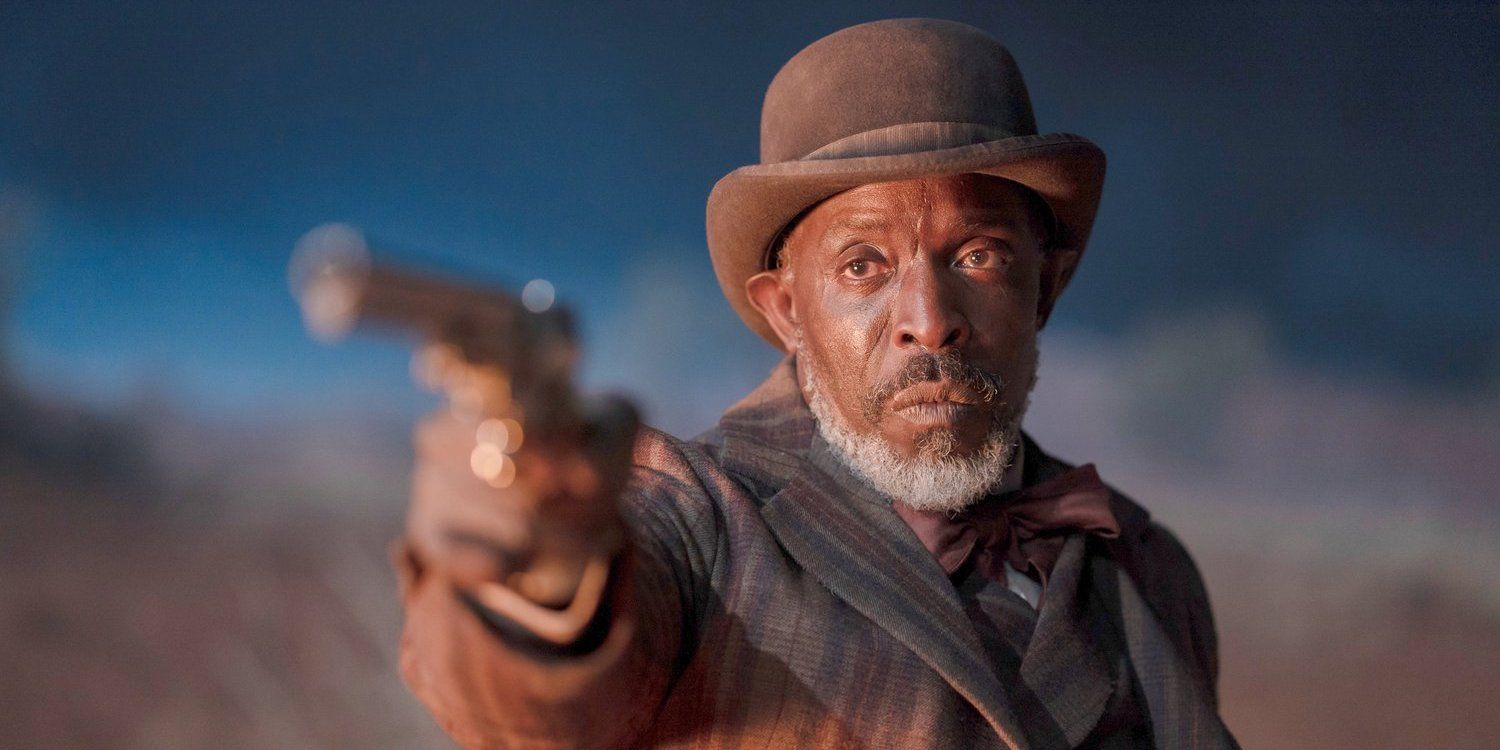The image captures a dramatic still from a Western movie featuring an African American man in his sixties, his intense demeanor highlighted by a prominent scar running from the middle of his forehead down the right side of his nose and cheek. He sports a grayish-white beard paired with a darker brown mustache. He wears a dark brown, old-fashioned bowler hat with curled edges, alongside a tan jacket adorned with darker reddish-brown stripes, and a brownish bowtie. The man is poised to fire, holding a pistol in his right hand with a gold ring visible on his middle finger. His focus is directed just to the right of the camera. The background, a blurred mix of dark blue sky and possibly desert or mountainous terrain, suggests an outdoor nighttime scene.